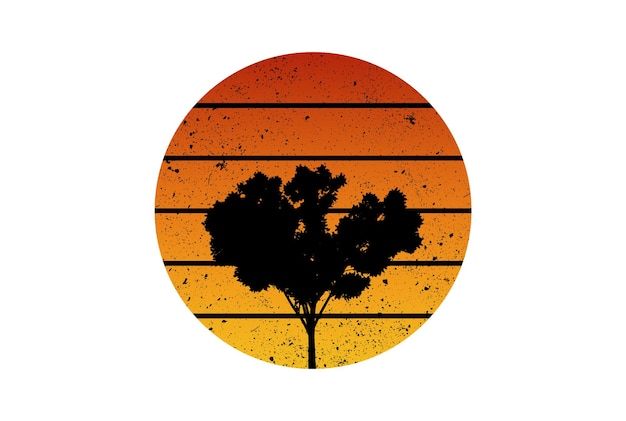This illustration features a circular design that captures the essence of a sunset sky. The background transitions from a deep, dark orange at the top to a lighter orange and yellow towards the bottom, creating a vivid gradient reminiscent of a setting sun. The circle is evenly segmented by five horizontal black lines, with some lines intersecting the central silhouette of a bushy, deciduous tree. This tree, entirely black in silhouette, has a thin trunk that splits into a Y-shape with branches spreading out, adorned with foliage resembling spiky cotton balls. Adding texture to the image, there is a speckly pattern of black dots and smears, primarily concentrated at the top and towards the sides of the circle. The meticulous details and dynamic colors within this circular frame evoke the tranquil beauty of a sunset landscape.